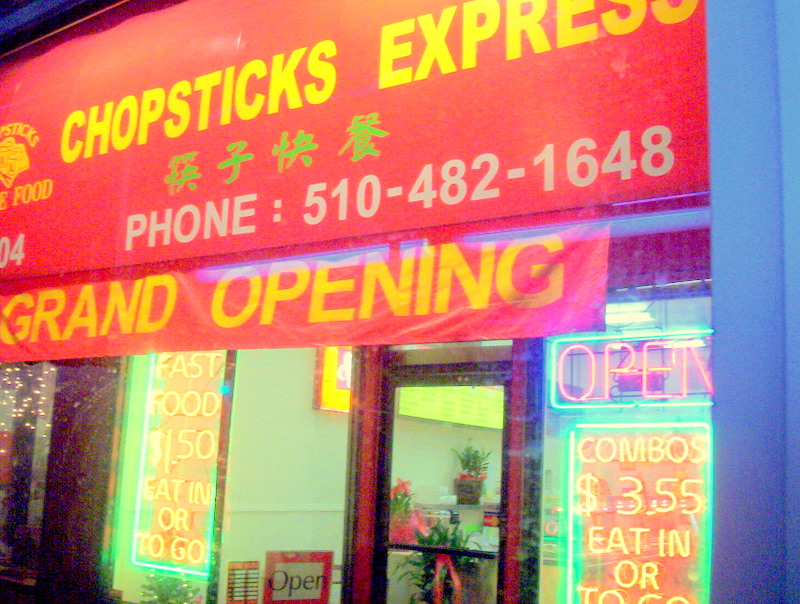The image captures a vibrant and colorful storefront of the Chopsticks Express restaurant, taken at night. Dominating the top of the scene is a large, red banner with "Chopsticks Express" prominently displayed in bold, yellow, all-caps letters, flanked by four green Oriental symbols. The banner also features the phone number "510-482-1648" in white text, suggesting the establishment is located in the United States. A secondary, bright red banner hangs below, announcing the "Grand Opening" in large, yellow letters.

The storefront window is illuminated by various neon signs. On the left window, a neon sign advertises "Fast Food $1.50, Eat In or To Go" in white lettering. The window also features a bright neon "Open" sign outlined in blue, indicating that the restaurant is currently open. To the right, another neon sign reads "Combos $3.55, Eat In or To Go" in yellow text. The front entrance includes a glass door framed by black and red trim, with white pillars on either side and a red horizontal support above. Inside the door, additional fluorescent lights further highlight the restaurant's offerings and business hours.

Despite the blurriness, the photo’s rich color palette and the mix of lit signage communicate a welcoming, bustling atmosphere ideal for diners seeking quick and flavorful meals.